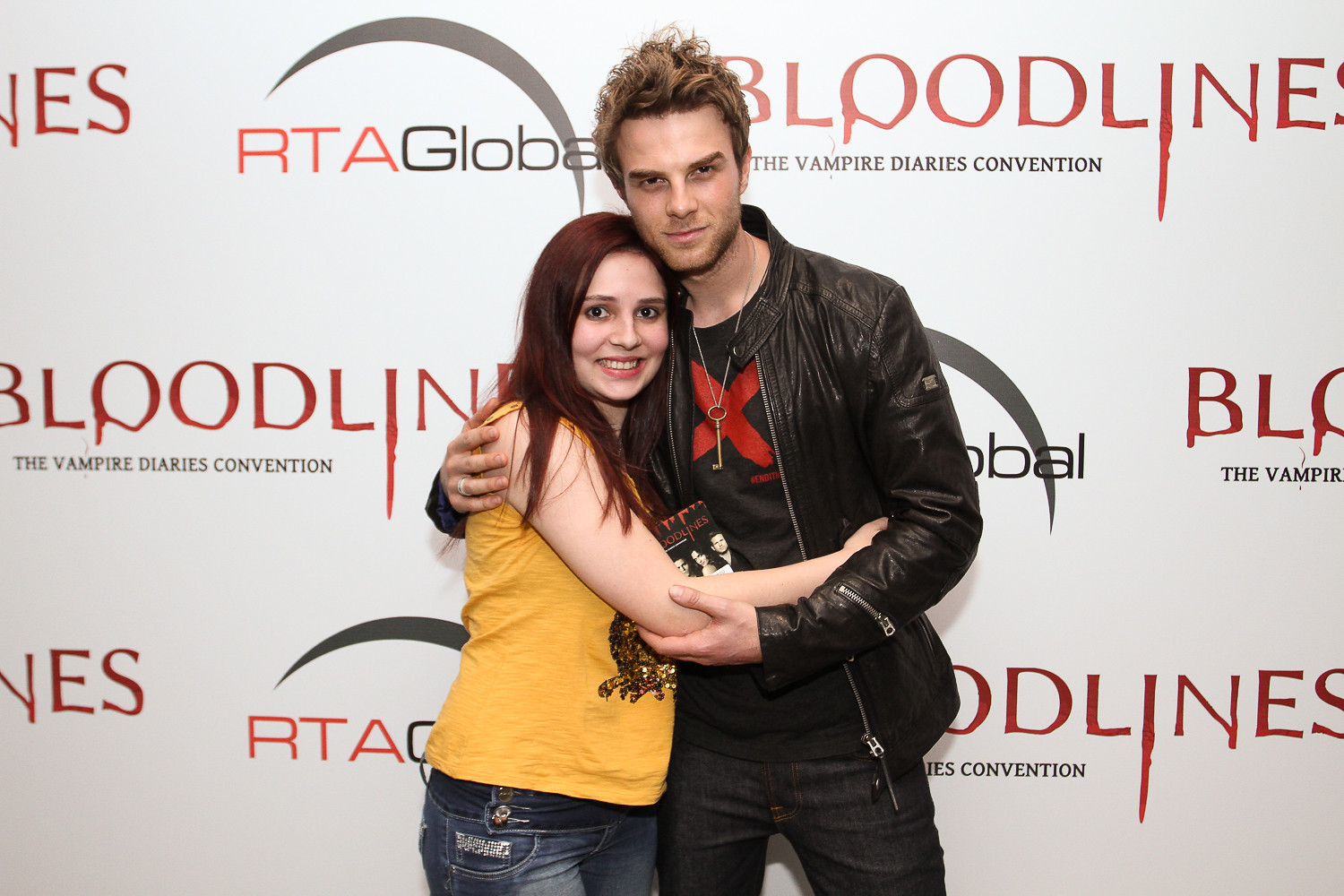In front of a backdrop that reads "Bloodline, the Vampire Diaries Convention" and "RTA Global," a young man and woman pose closely together. The man, sporting short brown hair, is dressed in a black and red T-shirt with an X design, a leather jacket with silver zippers, and dark jeans. He also wears a chain necklace with a gold key and has a ring on the third finger of his right hand. The woman, with long reddish-brown hair cascading past her shoulders, is clad in a sleeveless yellow shirt and blue jeans with silver detailing. She appears excited and a bit in awe, smiling broadly, while the man has his arm wrapped around her in an affectionate gesture, possibly indicating their roles as fan and actor in the convention setting.